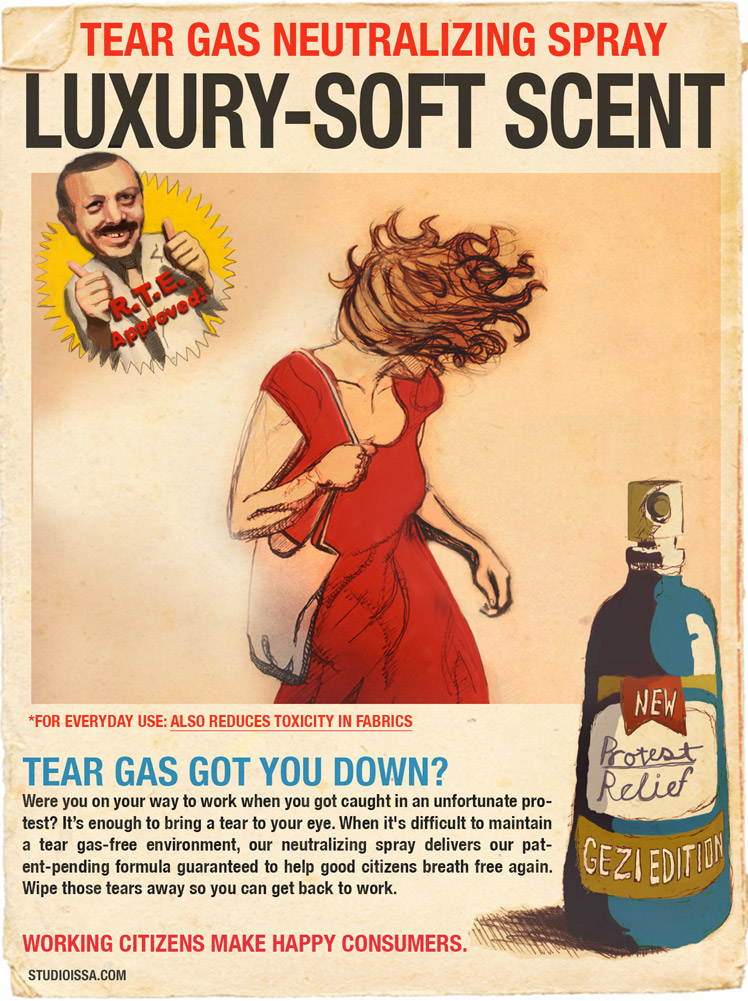The image appears to be a satirical magazine advertisement for a product called "Tear Gas Neutralizing Spray" with a "Luxury Soft Scent." The background mimics weathered paper, giving it an old-school feel. Prominently displayed across the top in red and black type, the text reads: "Tear Gas Neutralizing Spray, Luxury Dash Soft Scent."

In the upper left corner, there's a caricature of an Arabic man with a bushy beard, depicted with a large head and small body, giving two thumbs up inside a yellow circle, accompanied by the label "RTE Approved." The central figure in the advertisement is a drawing of a woman in a red dress, her red hair dramatically flying in all directions, suggesting distress or agitation.

Towards the bottom right, the ad features a drawing of the spray bottle itself, branded as the "New Protest Relief Gezi Edition." Text alongside the bottle claims, "For everyday use, also reduces toxicity of fabrics," and poses the question, "Tear gas got you down?" The advertisement humorously assures potential users that the spray will help them handle the effects of tear gas, stating, "Our neutralizing spray delivers our patent-pending formula guaranteed to help good citizens breathe free again. Wipe those tears away so you can get back to work." It concludes with the tagline, "Working citizens make happy consumers," and a reference to the website "studioissa.com."